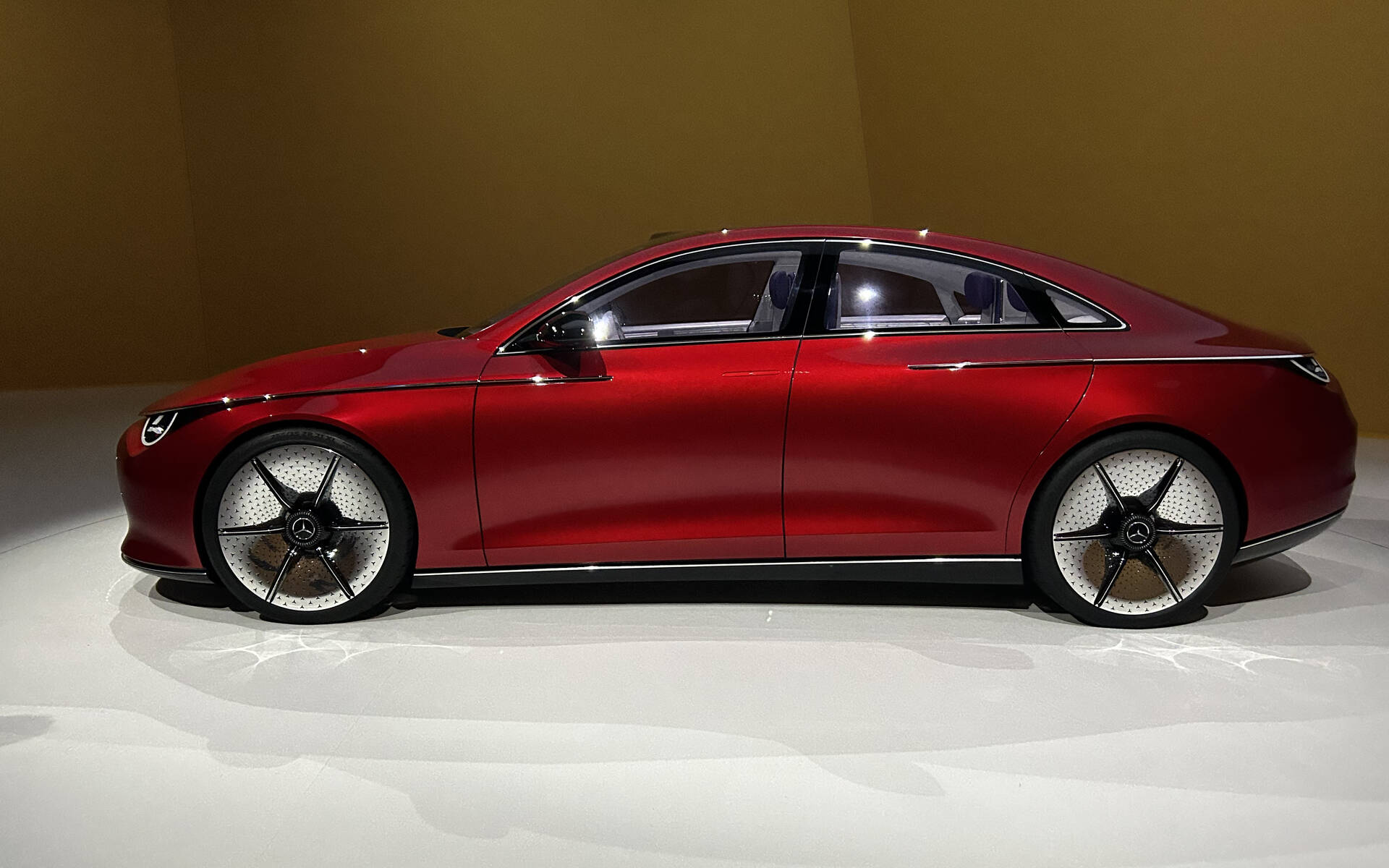The image showcases a sleek, cherry-red Mercedes-Benz on display in a showroom with a glossy white floor and a gold-colored wall. The car features a distinct, aerodynamic design with a sloped roofline and electronic, two-door access. Its unique wheels are black with six stylish spokes and intricate white patterns between them, creating an interesting effect. Notable details include black trim around multiple windows, black side mirrors, and a gray and silver accent along the rocker panels. The shiny red exterior captures the overhead light, adding to its striking appearance in the well-lit showroom.